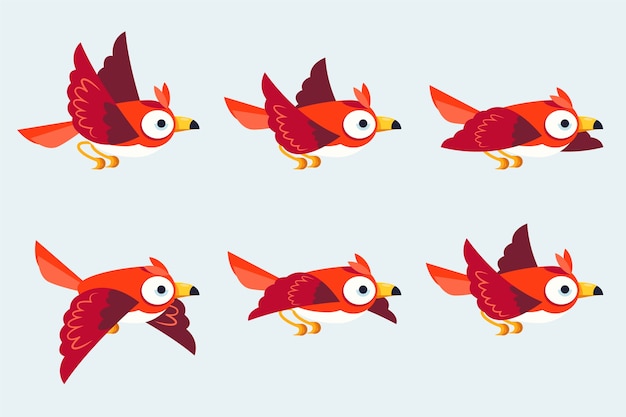The image depicts a cartoon representation of six birds arranged in two rows and three columns on an off-white or light gray background. Each bird, identical in design, is flying with red-toned bodies and distinctive features. They all face towards the right with their wings in various positions—some wings are raised upwards while others are down or stretched out to the side. The birds are characterized by their large, white circular eyes with black pupils, accompanied by hints of blue, and two small feathers on top of their heads. Their yellow beaks have black tips, and their legs are tucked underneath their round bodies. The birds display a gradient in their plumage with brighter orange upper parts and lighter orange or white lower parts. The tail feathers are light orange on the underside and vivid orange on the top. The wings exhibit a range of red shades, from bright red to burgundy, contributing to the dynamic and lively portrayal of these animated birds.